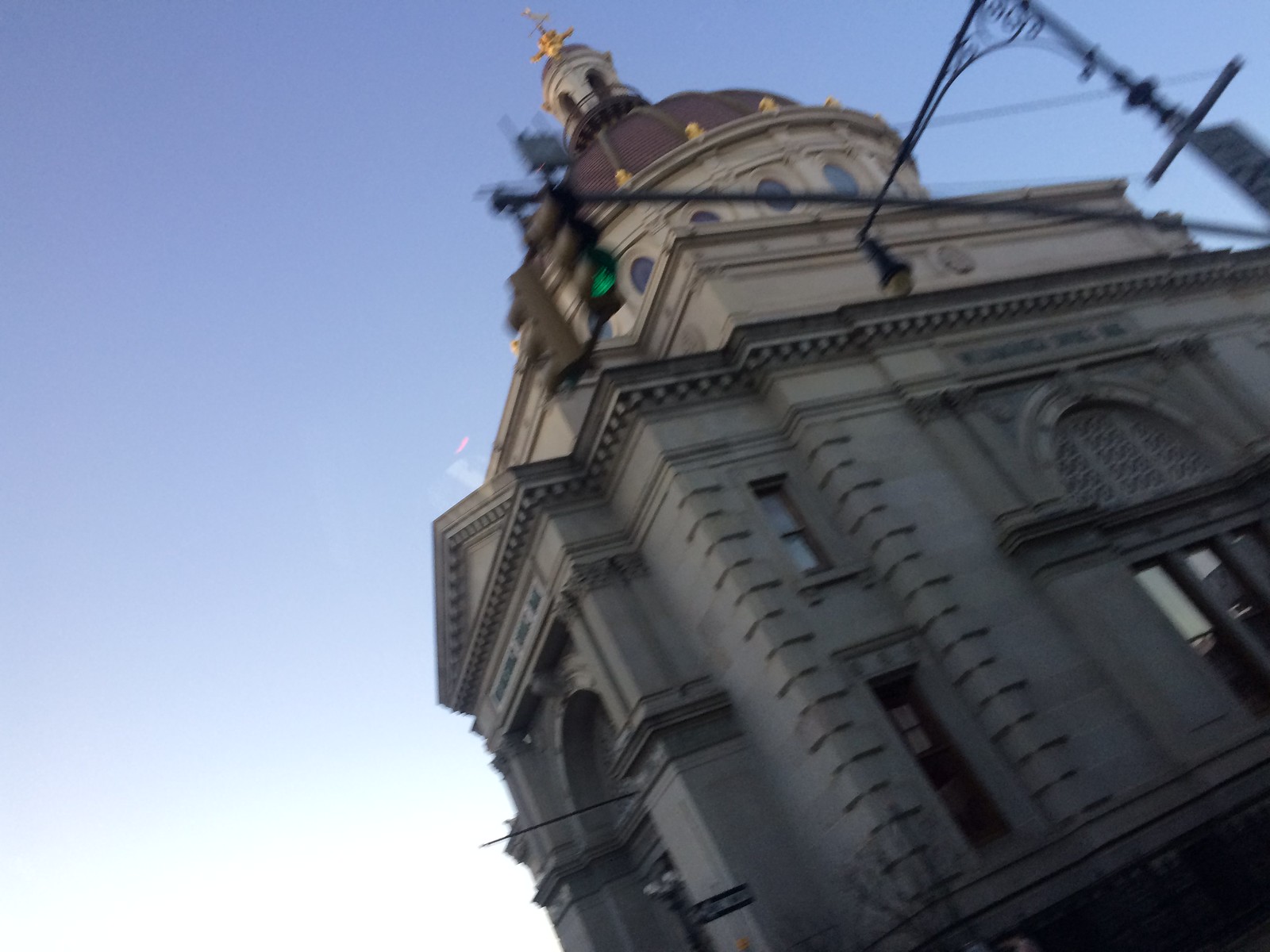The photograph depicts a blurry image of a state or federal public building, identified as the Wyoming City Hall, captured from a lower diagonal angle, looking up as though taken from a kneeling position. The building, predominantly tan stone, features intricate Gothic architecture with ornate stonework and numerous arches over the windows and entrances. It boasts a striking dome made of red tiles adorned with a golden pinnacle at its peak. This dome, surrounded by equally spaced golden structures along its circular outline, adds grandeur to the building’s design. The image is slightly obscured by a green stoplight and a wrought iron street lamp with a curled design in the top right corner. Additionally, the bottom of the photo reveals a leafless tree and another street lamp against a clear, blue, cloudless sky.